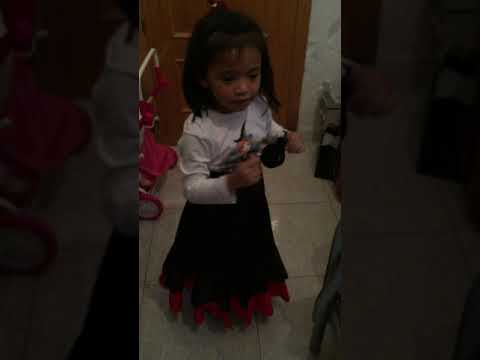In this low-quality, pixelated vertical photograph, a young girl around four years old is standing inside a house on a light, white-tiled floor. She has long black hair and is dressed in a white long-sleeved blouse, paired with a floor-length black skirt that has red fringes along the bottom. Her expression is neutral, possibly caught mid-moment while showcasing her toys. In her hands, she holds a small witch toy and another unidentified object. The background reveals a pink and white stroller and a wooden door. The image's dim lighting makes it difficult to discern whether it was taken during the day or night.